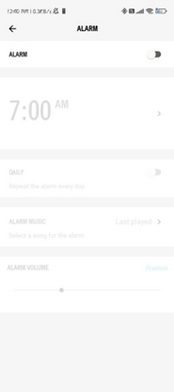The image is a blurred photo taken from a cell phone displaying the alarm settings screen. The top portion contains a light gray rectangle that contrasts with a dark section on the upper left. Within this rectangle, the time seems to be 12:40 PM, though it is difficult to discern clearly. In the top right corner, faint icons indicate signal strength, Wi-Fi, and battery life, all hard to make out due to the blurriness.

On the left side, a bell icon with a line through it shows that the alarm is off. Directly next to the time, a dark black left arrow is visible. Centrally positioned within the gray rectangle, the word "ALARM" is boldly displayed in all capital letters.

Below this, the screen transitions to a white background where the word "Alarm" is written in black on the left. Adjacent to it on the right is a slider switch with a white circle positioned to the left, indicating the alarm is deactivated. Further down, another shaded section reveals text reading "7:00 AM" with a right-facing arrow beside it. Underneath, a line of text states "Daily" followed by a note about repeating the alarm every day, though details remain obscured.

Further sections vaguely show options for "Alarm Music," where users can select a song for the alarm, marked by a black right-facing arrow, and "Alarm Volume," both of which are also shaded out and difficult to read clearly.